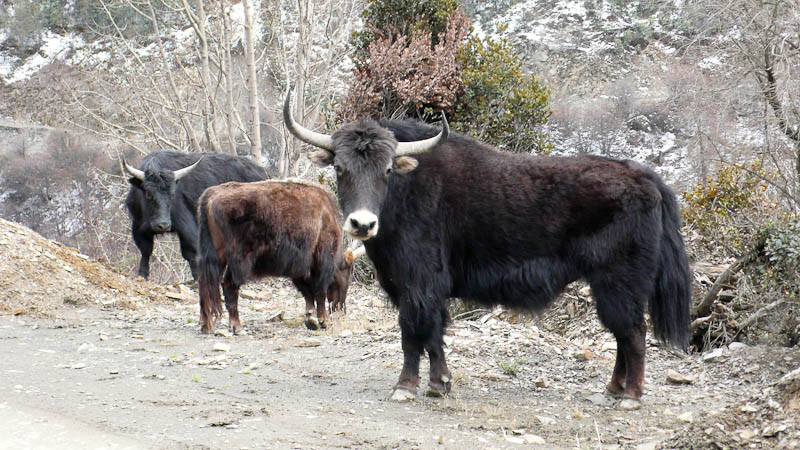The color photograph captures a rugged, barren hillside in a wild, outdoor setting. The landscape-oriented image prominently features three bovine animals, possibly wild cows or oxen, distinguished by their long, curved ivory-colored horns that extend from the sides of their heads and then curve upwards.

In the foreground, on the right side of the frame, stands a dark brown cow with a nearly black coat stretching along most of its body and a black horse-like tail. It faces the camera with a white muzzle and ears sticking straight out, while its body is positioned side-on.

Behind this cow, two more animals are visible: one in the far background appears almost entirely black, while the other, situated in the middle, is a lighter brown with some darker patches. This middle cow is seen bending down, possibly eating something off the ground.

The setting is a steep, slick hillside covered in thin grey gravel, with sparse, dead vegetation and twigs scattered about, contributing to the scene's desolate feel. In the distance, another rocky hillside rises, reinforcing the harsh, rugged terrain. Trees with green leaves and some with dead or no leaves add sparse color variations to the background. The natural setting and the serene, yet somewhat stark, pastoral life of these majestic animals are vividly captured in this striking photograph.